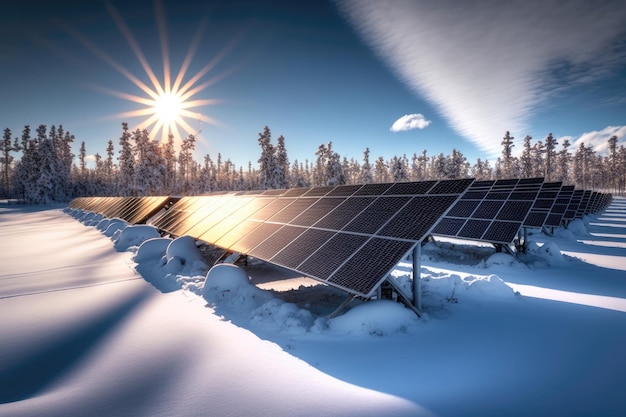A captivating image showcases an expansive field of solar panels, meticulously aligned and tilted at an angle on a support system. The solar panels are surrounded by a snowy landscape, with no snow visible on the panels themselves. In the foreground, the windblown snow exhibits a textured surface, and rough snow accumulation is seen at the base of each panel, as though it has melted off them. The top third of the image features a vivid blue sky with patches of white, fluffy clouds concentrated on the right side. Dominating the left third of the sky is a bright sun, radiating sharp, distinct rays. Along the horizon line, a series of evergreen or pine trees stands, their snow-capped branches glowing faintly yellow from the sun's light. This potentially AI-generated scene captures a serene winter moment, blurring the line between reality and digital artistry.